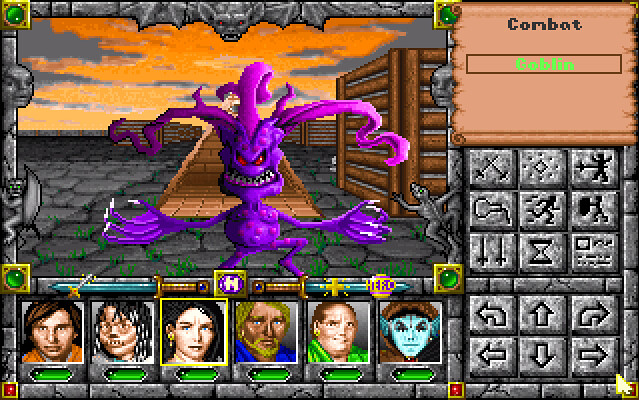The image depicts a scene from a video game featuring a menacing, purple goblin staring directly at the screen. The upper-right corner of the screen displays the title "Combat Goblin," accompanied by various symbols and instructions for combat. The backdrop showcases an eerie setting with an orange sky and black tiled bricks covering the ground. To the right of the goblin, a fence adds to the scene's ominous atmosphere. Below the central image, there are six different characters available for the player to choose from, presumably to assist in battling the goblin.